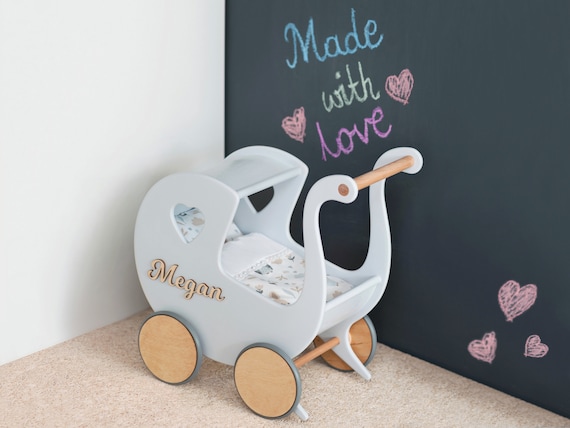This image showcases a quaint and charming scene featuring a wooden toy stroller predominantly painted in white, nestled in the corner of a cozy room. The stroller boasts four wheels, each crafted from natural wood and adorned with a delicate gray rim. The wooden handle and structural elements of the stroller add to its rustic charm. On the side of the stroller, the name "MEGAN" is elegantly displayed in gold letters.

The wall to the left of the stroller is a plain white, while the wall on the right contrasts sharply with its chalkboard-like appearance in black. Etched on this black wall, in vibrant chalk colors, is the phrase "MADE WITH LOVE" – "MADE" in blue, "WITH" in green, and "LOVE" in pink. Accompanying this heartfelt message are five pink heart drawings, with two hearts flanking the text and three hearts positioned at the bottom right corner.

Inside the stroller, a soft white blanket adorned with subtle animal designs provides a cozy touch, suggesting a space meant for play and comfort. The room itself has a beige floor, emphasizing the warm and inviting atmosphere. The overall setting is enriched with thoughtful details that evoke a sense of loving craftsmanship and childhood nostalgia.